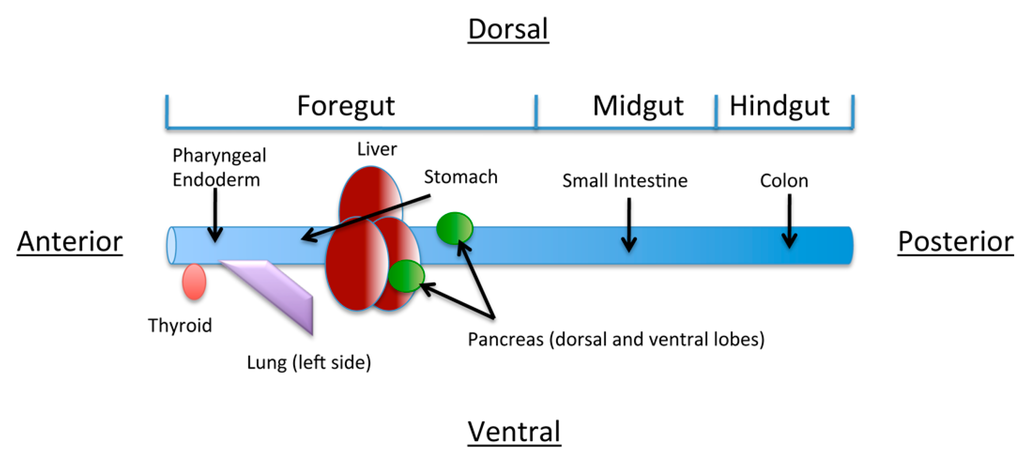This detailed medical diagram illustrates the anatomical layout of the human digestive and endocrine systems along the body’s dorsal-ventral axis. It features a prominent vertical blue tube symbolizing the gut, which runs from the dorsal (top) to the ventral (bottom) with labels at its extremities. The diagram is sectioned into three main regions: foregut, midgut, and hindgut.

1. **Foregut Region:** 
   - **Thyroid:** Positioned at the anterior-most point and indicated by a pink oval.
   - **Pharyngeal Endoderm:** Directly above the thyroid, marked at the top left.
   - **Liver:** Located centrally with three large red ovals representing it.
   - **Stomach:** Situated next to the liver, with an overarching label.
   - **Pancreas:** Displayed as two green circles denoting the dorsal and ventral lobes, nestled around the liver and stomach areas.

2. **Midgut Region:**
   - **Small Intestine:** An arrow points from this section towards the blue tube, indicating its connection.

3. **Hindgut Region:**
   - **Colon:** Labeled under this section, with an arrow leading to the blue tube.

Additionally, the diagram has spatial cues:
- **Anterior (left)** and **Posterior (right)** are labeled to orient the viewer.
- The **Left-side Lung** is highlighted as a purple trapezoid branching off from the tube.

Meant as an educational tool, the diagram uses a combination of colored shapes (pink, green, red, and purple) and black text on a white background to depict and label significant organs and structures within these regions.